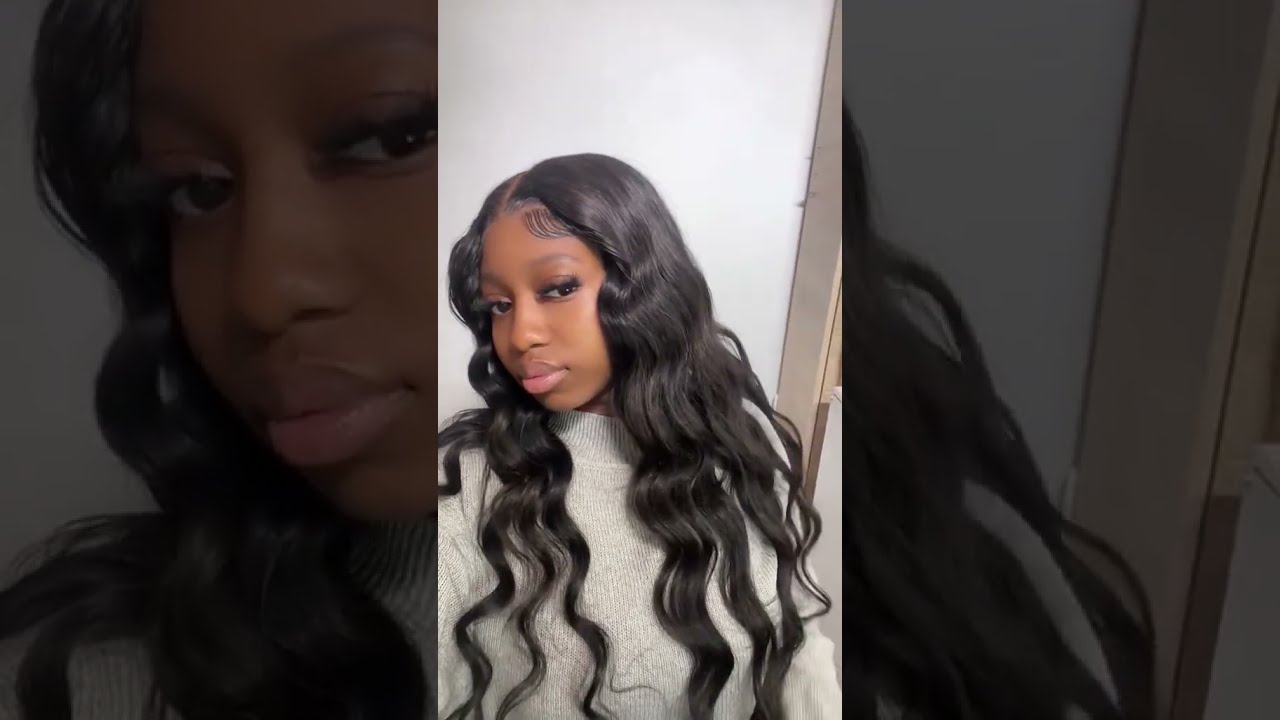This vertically-oriented image is a triptych featuring a young black woman, likely in her teens or early 20s, with strikingly long, wavy black hair that cascades down to nearly her waist. The centerpiece shows her well-lit face in high detail, with her head slightly tilted towards her right shoulder, giving a soft, contemplative look slightly to her left. She is adorned in a light gray turtleneck sweater and has meticulously styled baby hairs pressed against her forehead in a wave-like pattern. The backdrop consists of a plain white wall, with the faint outline of a doorway frame on her right side. On the left and right sides of the collage are close-up, zoomed-in sections of the main image. The left zoom-in focuses on her facial features and the left side of her wavy hair, while the right zoom-in emphasizes the luxuriant texture and length of her hair. The unified composition highlights her serene expression, detailed styling, and voluminous hair, suggesting that the photo might be a selfie intended for social media or a makeup tutorial.